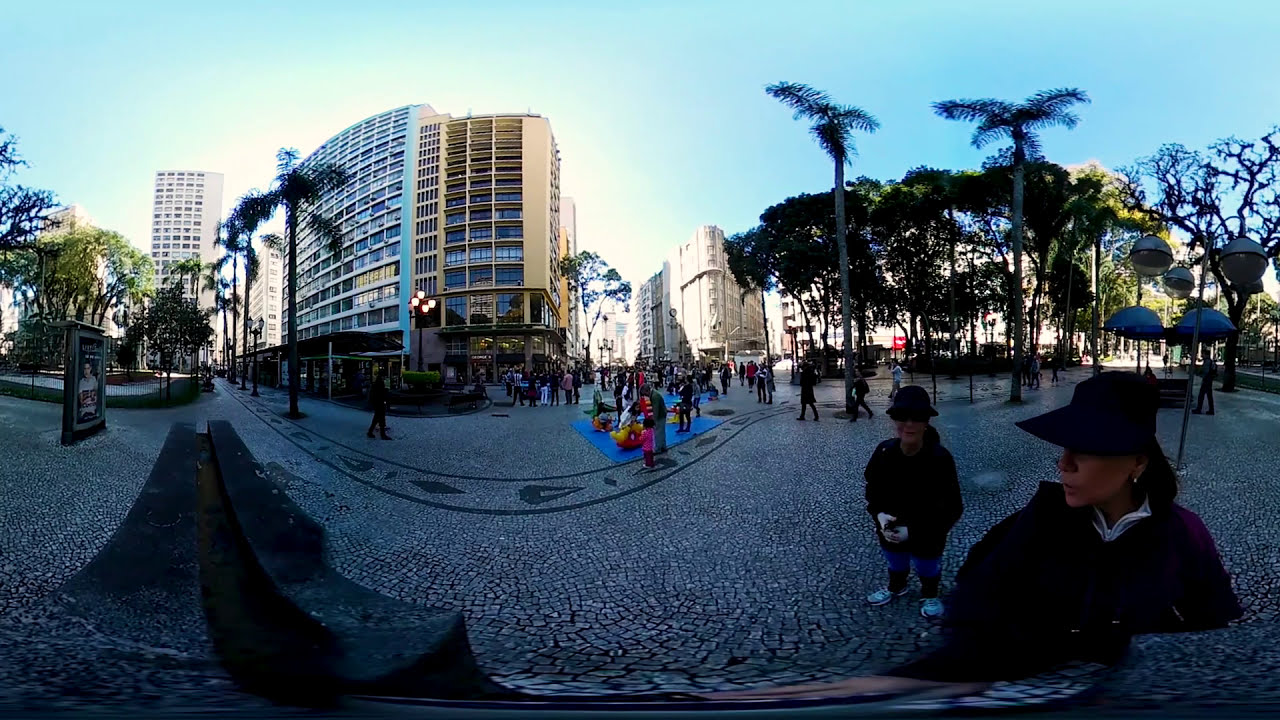This outdoor photograph captures a bustling urban courtyard with a distinct curvature, possibly due to panoramic or fisheye distortion. The ground is paved with small, uniformly shaped grey and green bricks arranged in detailed patterns, including some diamond shapes. At the center of the courtyard, there is a children's play area. Numerous people are walking about, enjoying a sunny day under a clear blue sky.

In the foreground, two individuals stand out. One wears a black hat, black jacket, and long pants, and another is identifiable by white tennis shoes and a white shirt collar peeking out from a black jacket. In the background, towering high-rise buildings, likely apartments or condominiums, frame the scene alongside a hotel. Palm trees and other greenery add a touch of nature. The sunlight casts a warm glow, though some people are dressed in jackets, suggesting mild weather. Interesting sculptures or light fixtures decorate the street, adding to the urban charm.